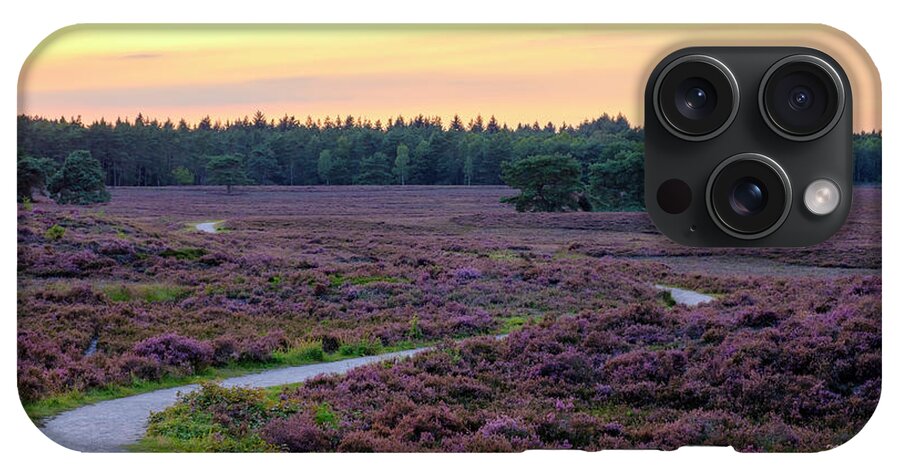This image shows the back of a smartphone encased in a decorative cover designed for an iPhone. The cover features an exquisite nature scene: a field of vibrant purple and violet flowers, identified as lavender, interspersed with patches of grass. A small, winding stream snakes through the lavender field, its serpentine path curving gently down a hill, occasionally peeking through the dense flower cover. On the right side of the image, adjacent to the phone's camera lenses—which include three large lenses for photos, a black eyepiece-like feature possibly for measuring brightness, and several white elements likely functioning as a flash—there is a grove of trees. In the far background, a large forest of pine trees creates a serene backdrop under a sky painted in hues of yellow and purple. The phone case itself is displayed horizontally against a blank background, emphasizing its detailed and picturesque design.